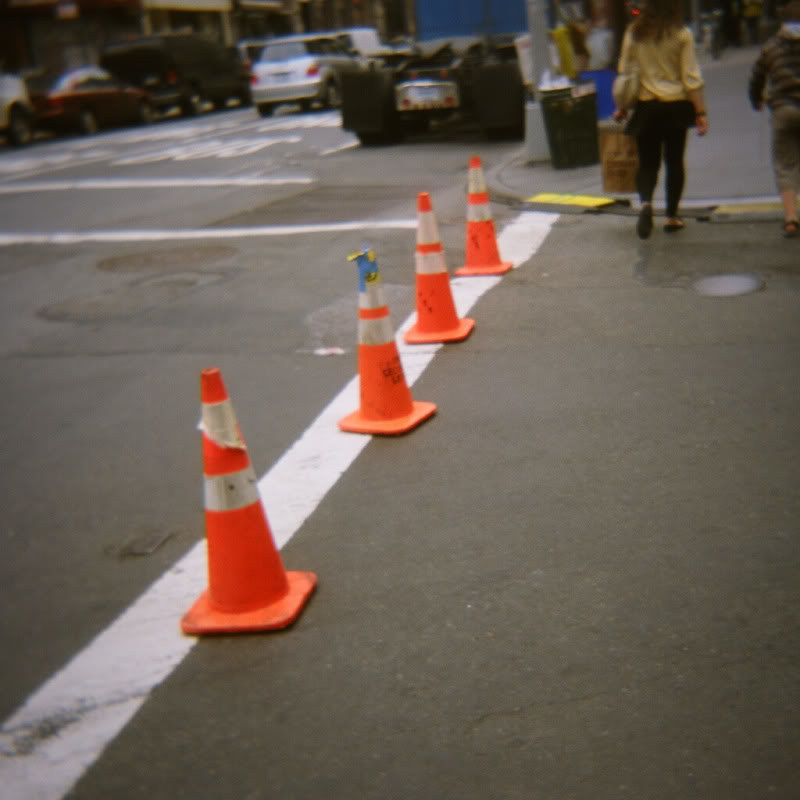The image captures a bustling urban street scene. At the center, four orange traffic cones are aligned on the road, likely marking some construction or maintenance work. On the right side, although the crosswalk lines are not visible, pedestrians can be seen crossing the street. Among them stands out a person with auburn hair, dressed in a yellowish-gold top, black leggings, and sandals, heading towards the sidewalk. This sidewalk features a yellow tactile paving rectangle, designed for visually impaired individuals, leading onto a gray pavement. Adjacent to the sidewalk, a pole and a trash can are also visible. On the left side of the image, a white or gray car is driving along the street, which is marked with white lane lines and some partially obscured white text. The overall scene illustrates a typical moment in a busy city environment.